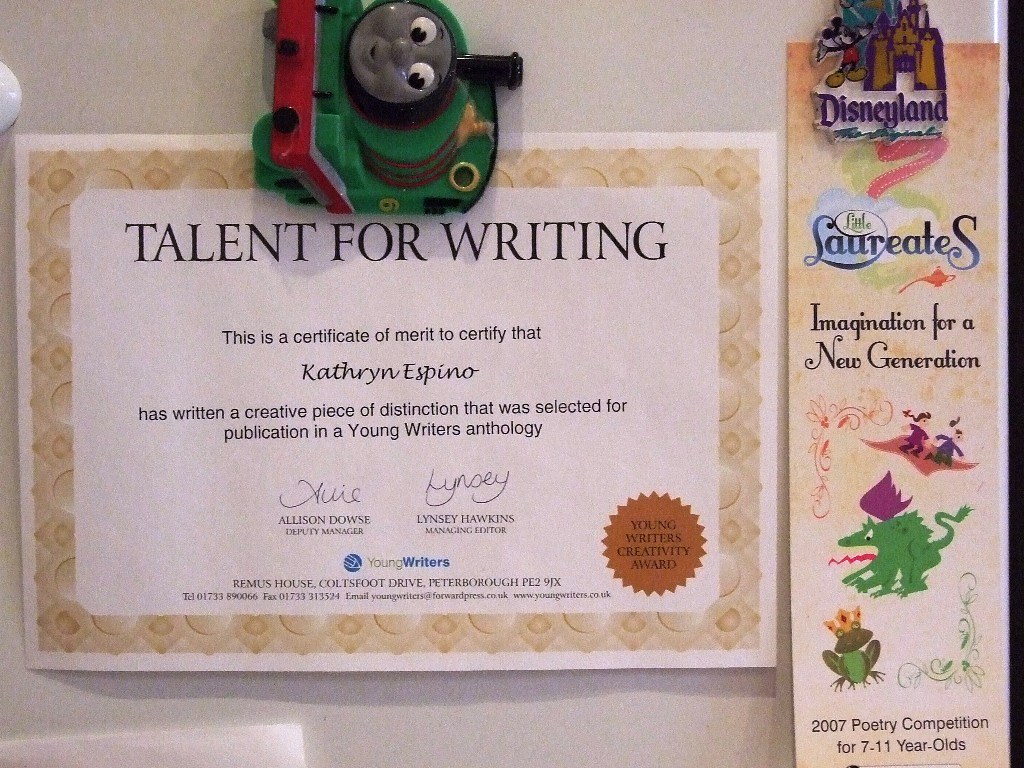In this detailed refrigerator display, a talent certificate of merit dominates the scene, recognizing Catherine Espino for her exceptional creative piece selected for publication in the Young Writers Anthology. The certificate reads: "This is a certificate of merit to certify that Catherine Espino has written a creative piece of distinction that was selected for publication in the Young Writers Anthology." It includes signatures from Alison Dowes, Deputy Manager, and Lindsay Hawkins, Managing Editor, along with a seal that reads "Young Writers Creativity Award." Thomas the Train character magnet holds the certificate in place.

To the right, a colorful Disneyland magnet secures a bookmark-like flyer that announces the "Little Laureates Imagination for a New Generation, 2007 Poetry Competition for 7 to 11-year-olds." The drawing on the bookmark features whimsical images of a dragon, a frog, and some children, adding a lively touch. The refrigerator, adorned with magnets and awards, bursts with an array of colors, including green, red, gray, purple, gold, blue, white, and black, emphasizing a vibrant and creative household where children's achievements are proudly displayed.